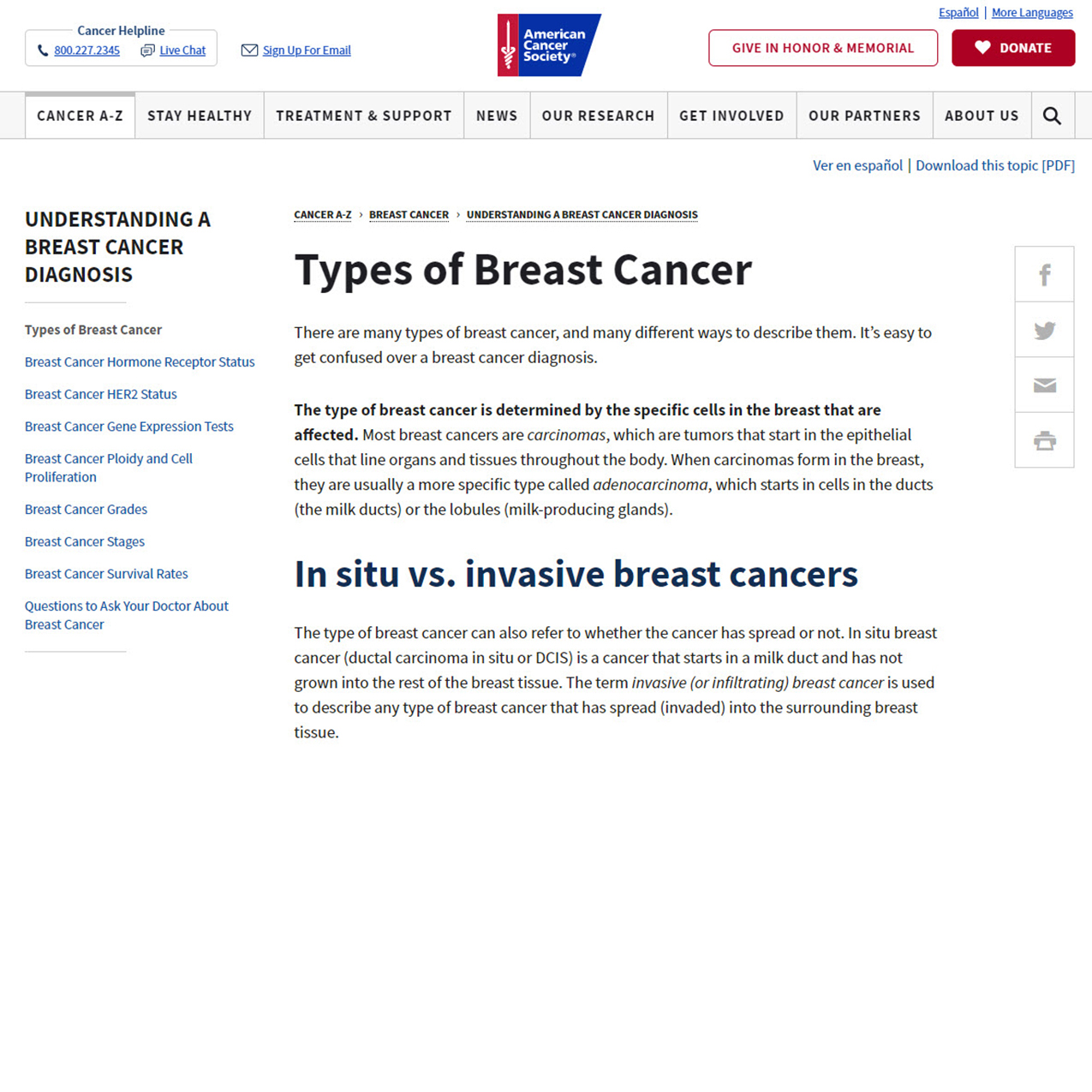The image is a screencap from the American Cancer Society's website. At the top center, there's a logo composed of a blue square with a red left side, featuring a white stick figure with a circular or tornado-like effect on the right. The logo text, "American Cancer Society," is written in white against the blue background.

In the top left corner, there are navigational links in blue text: "Career," "Cancer Helpline," a phone number (which is not clearly visible), "Live Chat," and "Sign Up for Email." On the top right, there are two buttons: the left one is a white rectangle with red text that reads "Give in Honor and Memorial," and the right one is dark red with white text that reads "Donate" accompanied by a white heart icon. Above these buttons, "Español" and "More Languages" are also in blue text.

Directly below this top section, a navigation bar spans the width of the page with links in the following order: "Cancer," "Stay Healthy," "Treatment & Support," "News," "Our Research," "Get Involved," "Our Partners," and "About Us." A magnifying glass icon, presumably representing a search function, is located on the far right of this bar.

Beneath it, there are small blue text links, "Ver en Español" and "Download this Topic PDF." Moving further down, the left sidebar contains a section titled "Understanding a Breast Cancer Diagnosis" with several subsections listed below. These subsections include: "Types of Breast Cancer," "Breast Cancer Hormone Receptor Status," "Breast Cancer HER2 Status," "Breast Cancer Gene Expression Test," "Breast Cancer Ploidy and Cell Proliferation," "Breast Cancer Grades," "Breast Cancer Stages," "Breast Cancer Survival Rates," and "Questions to Ask Your Doctor About Breast Cancer." Each subsection title is in blue text.

In the main body of the website, small black text labels the section as "Cancer, a Disease, Breast Cancer, Understanding a Breast Cancer Diagnosis." The prominent heading "Types of Breast Cancer" follows, with explanatory text below explaining the various types and the specifics of a breast cancer diagnosis. There is a bolded statement that reads, "The type of breast cancer is determined by specific cells in the breast that are affected." The accompanying non-bold text details that most breast cancers are carcinomas, specifically adenocarcinomas, which start in the cells of the ducts and lobules.

Further down, another bold heading reads "In Situ vs. Invasive Breast Cancers." The text underneath explains the differences between these types, noting that ductal carcinoma in situ (DCIS) is a non-invasive cancer confined to the milk ducts, while invasive breast cancer refers to any cancer that has spread into surrounding breast tissue.

To the right of this main text, there are vertical buttons for social sharing and functions including Facebook, Twitter, email, and print, represented by gray icons. The website primarily uses black text on a white background, enhancing readability.